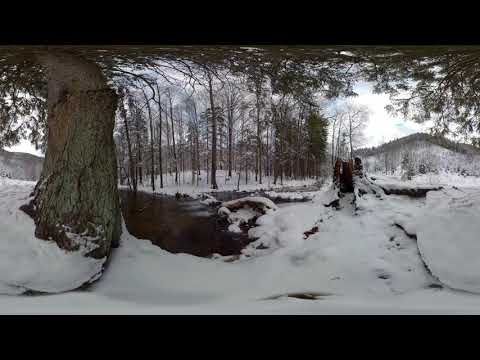This is a horizontally aligned rectangular 360-degree panoramic photograph capturing a serene, snowy nature scene. Dominating the left side is a thick tree trunk, accented by brown and green branches, extending upwards into a canopy of fir and pine needles. The ground is predominantly covered in snow, with some areas melted away revealing patches of dark, possibly watery, ground. The center of the image features a small wooden bridge, adding a focal point amidst the snow-covered landscape. Tall, thin trees, some with leaves and some without, form a backdrop that stretches into a mountainous area on the right. The white, mostly cloudy sky overhead enhances the tranquil ambiance, reflecting the diffused light throughout the scene. Despite the slightly warped appearance from the panoramic effect, the photo crisply captures the stillness of this undisturbed park, devoid of people or animals.